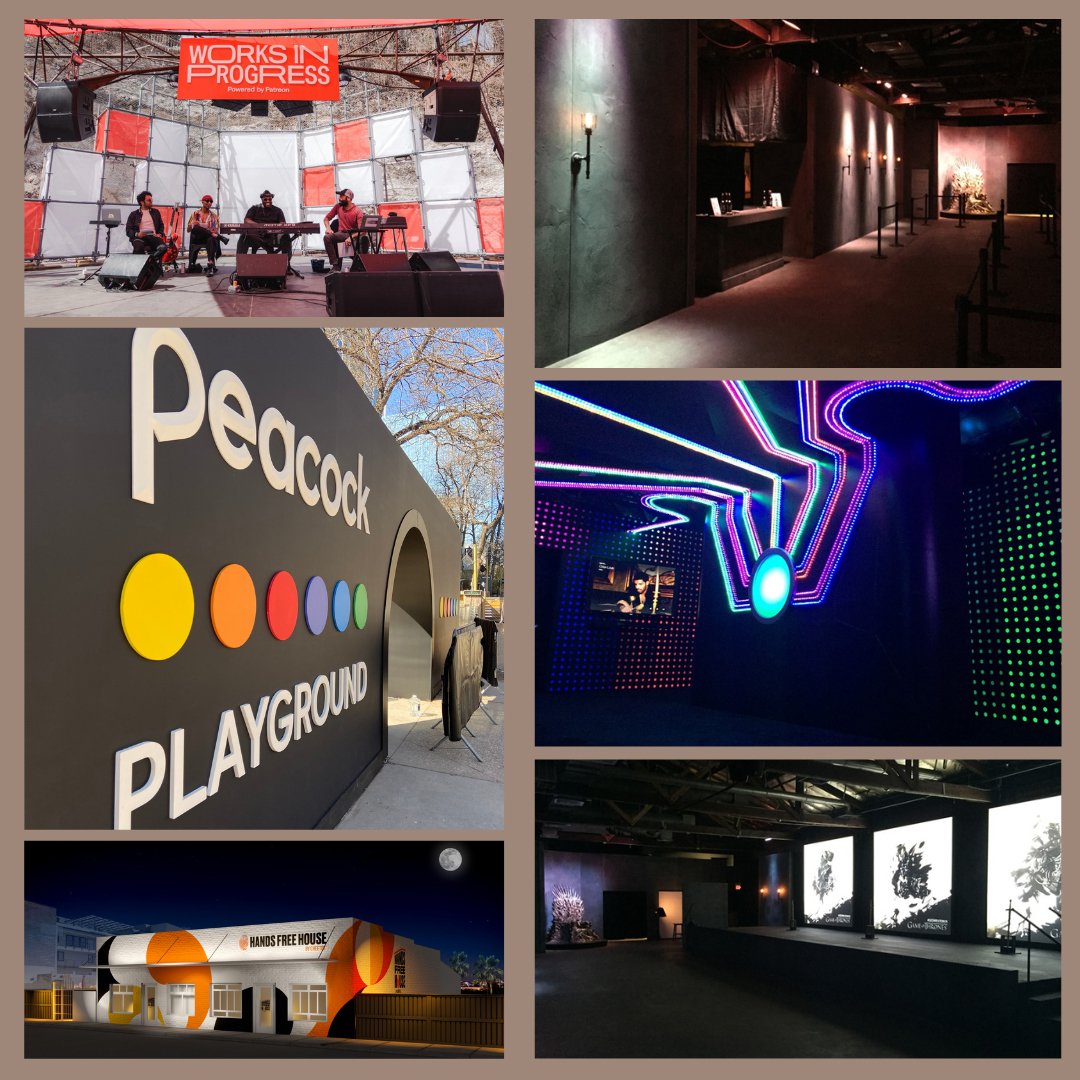The image is a collage of six distinct smaller pictures, each framed in a tan color. Starting from the top left, the first picture features four musicians performing in a studio with a red, gray, and white checkered background. At the top of this image, a red box displays the text "Works in Progress." Moving to the top center, there is a dimly lit hallway resembling a museum with dark gray walls and torchlight figures for illumination, and a path marked for visitors. The top right image shows another dark room, possibly a nightclub or studio, with vibrant wall lights and neon shapes, along with a television on the wall.

The middle left picture showcases a black background with the text "Peacock Playground," displaying circles in multiple colors: yellow, orange, red, purple, blue, and green, possibly representing a colorful outdoor tunnel with a tree in the background. The bottom left image depicts a white building with orange accents labeled "Hands Free House." Finally, the bottom right image seems to portray a dark stage area with what might be blobs or trees in the background and a small opening for a door, suggesting a stage setup in a dark room.